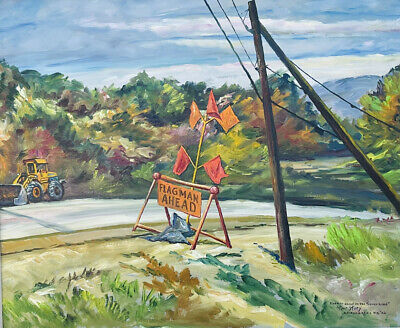This detailed illustration, created with visible pencil strokes, depicts a construction area set within a hilly, farm-like landscape. The scene features a roadway extending from left to right, bordered by green grass, lush open fields, and an array of vibrant trees exhibiting hues of green, yellow, and red-orange. On the upper side of the road, a yellow bulldozer (or backhoe) is actively engaged in excavation, its shovel digging into the earth and its black wheels and axles prominent. To the right side of the road, a triangular stand holds a sign reading "Flag Man Ahead," accompanied by five orange hazard flags. Nearby, a braced telephone pole, supported by another damaged pole, extends three wires across the area, indicating a recent break with the upper part of the pole bent and leaning. The detailed interplay of natural elements and construction activity provides a rich visual narrative of this outdoor scene.